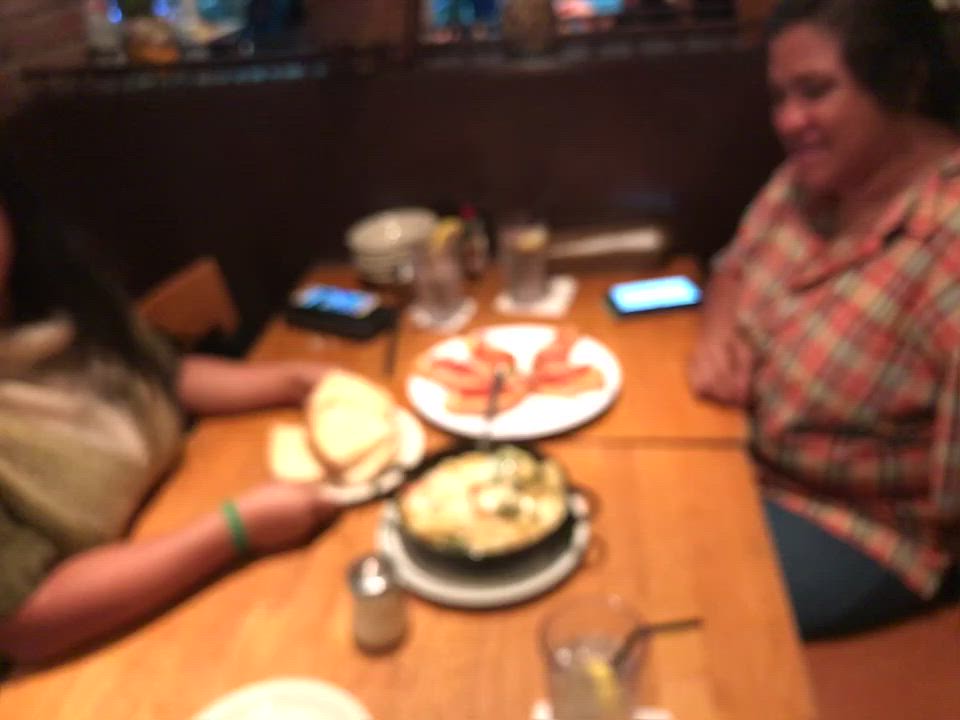This photograph, although very blurred, captures a cozy restaurant scene featuring two women seated at a double brown wooden table, with a brown wooden wall in the background. The woman on the left side of the table, partially cropped out of the image, wears a gray top and a green wristband on her right wrist. She holds a white plate with what appears to be a sandwich. Across from her, the second woman, with light brown skin, short black hair, and dressed in a red and tan plaid shirt and jeans, smiles warmly. Both women have their cell phones placed on the table in front of them, their screens faintly illuminated. The table is set with a variety of dishes, including a large white plate with five objects resembling appetizers, another white plate with a black bowl which might contain dip or soup, and a drink with a straw. Two water glasses with lemon slices, salt and pepper shakers, and a faint hint of colored lights or windows in the dark background add to the ambiance of this intimate dining moment.